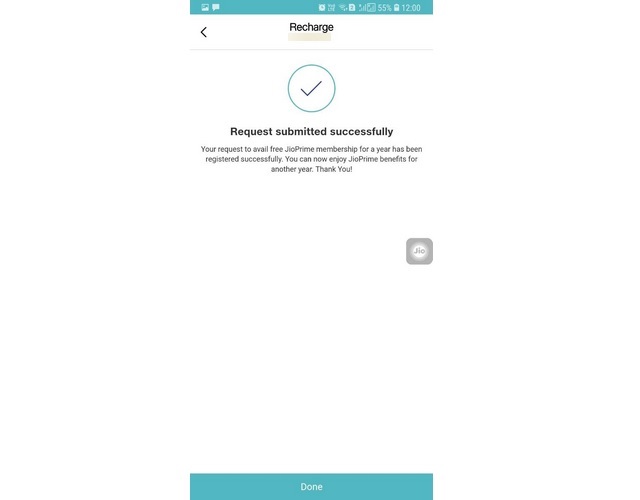A mobile device screenshot displaying a successful recharge confirmation is described in detail as follows: 

The screen has a small green bar at the top showing the time, 12:00, and a battery level indicator at 55%. The predominant background is white. At the top of the screen, there is a label with the text "Recharge" and a back button located to the left of it.

Below this header, there is a large check mark encased in a circle, symbolizing the successful completion of the process. Beneath this icon, the text reads, "Request submitted successfully." Further down, a smaller text elaborates, "Your request to avail free Jio Prime membership for a year has been registered successfully. You can now enjoy Jio Prime benefits for another year. Thank you."

Towards the bottom-right section of the screen, but slightly more towards the center, is the Jio logo, presented in gray with a white circle in its center. At the very bottom of the screen, there is a green button with white text that says "Done," indicating the next action the user can take by tapping it.